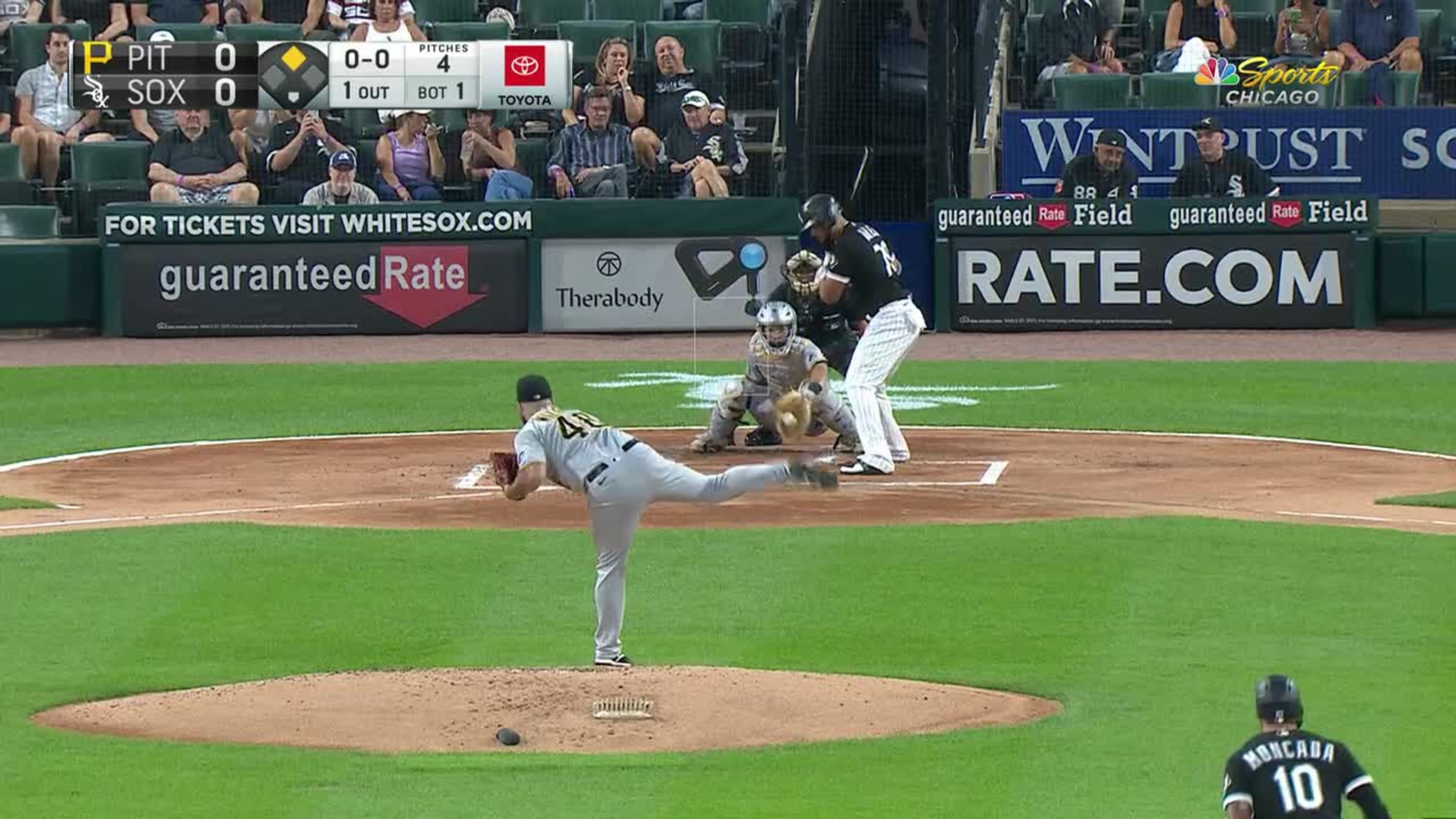The image captures a moment from a professional baseball game between the Pittsburgh Pirates and the Chicago White Sox, taking place at the White Sox's stadium. The scene is set in the bottom of the first inning with one out. A runner is leading off second base as the Pirates' pitcher, wearing a gray uniform with the numbers '48' visible and his leg in mid-air from the pitch, has just thrown the ball towards the catcher. The catcher, positioned behind home plate, is about to secure the pitch, which appears to be called a ball as the batter did not swing. 

In the background, the score is displayed in the top-left corner, showing 'PIT' for the Pirates and 'SOX' for the White Sox. The stadium is bustling with fans seated throughout, attentively watching the game. Surrounding the scene, various advertisements are prominently displayed. Directly behind the catcher against the wall, ads for 'rate.com' and 'TheraBuddy' are visible, along with a large Toyota banner above the scores. Additional text promoting ticket purchases is also visible, highlighting "visit whitesox.com" for more information. Coaches can be seen seated behind one of the ads, closely observing the game's progression and strategizing.